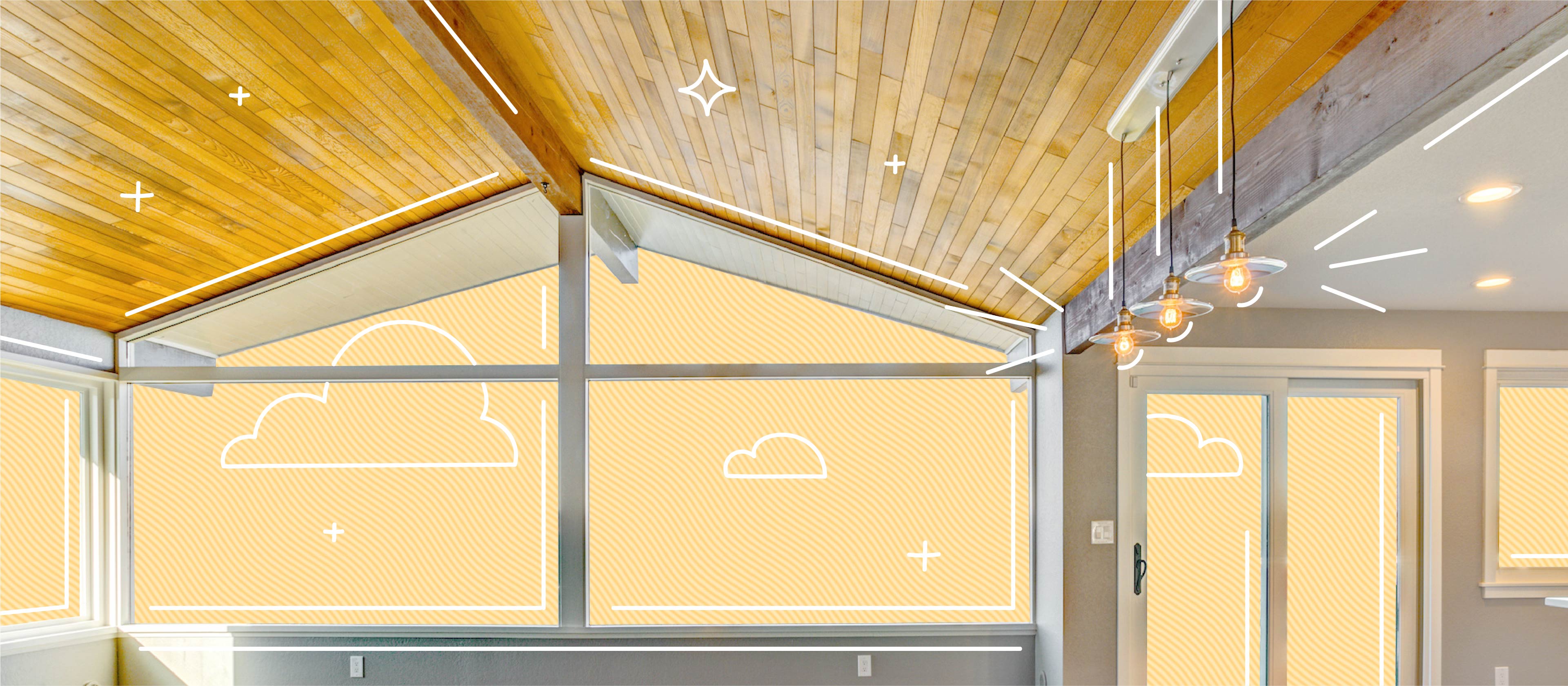A spacious room with a minimalist design is captured in a horizontal photograph, enhanced by digital artwork. The interior, painted in a medium gray tone, features a striking ceiling of attractive brown wooden slats, showcasing the wood grain, likely stained or polished. The room is dominated by large windows that constitute about 90% of the walls, allowing an abundance of light to flood in. These windows, formed by shapes of squares and triangles, open to a whimsical backdrop of a yellow sky adorned with simplistic, white, cartoon-like clouds and four-pointed stars, suggesting Photoshop edits. Hanging from the ceiling are three light fixtures, accentuated with white doodles of radiant lines. On the right side of the room, a sliding glass door reveals a glimpse into an adjacent space, which also seems to emit ceiling light. The blend of photographic realism and digital illustrations creates a unique, almost otherworldly ambiance, highlighting both the architectural elements of the showcase house and the playful, artistic embellishments.